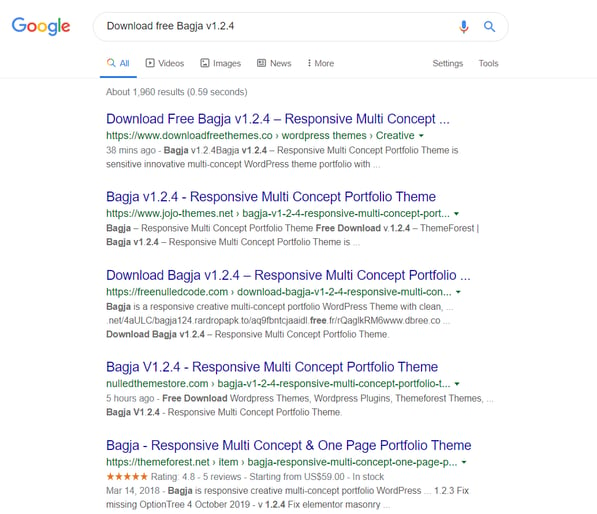This image depicts a Google search results page with a pristine white background. In the top left corner, the Google logo is prominently displayed, featuring a blue capital "G", a red lowercase "o", another yellow lowercase "o", a blue lowercase "g", a green lowercase "l", and a red lowercase "e". To the right of the logo, the search bar contains the query "download free by version 1.2.4 or Bagja", although the pronunciation of "Bagja" is ambiguous.

Below the search bar, there are various navigation tabs including "All", "Videos", "Images", "News", "More", "Settings", and "Tools". The search query has yielded approximately 1,960 results in 0.59 seconds. Within the visible portion of the screen, five search results are displayed, giving an indication of the content generated by the query.